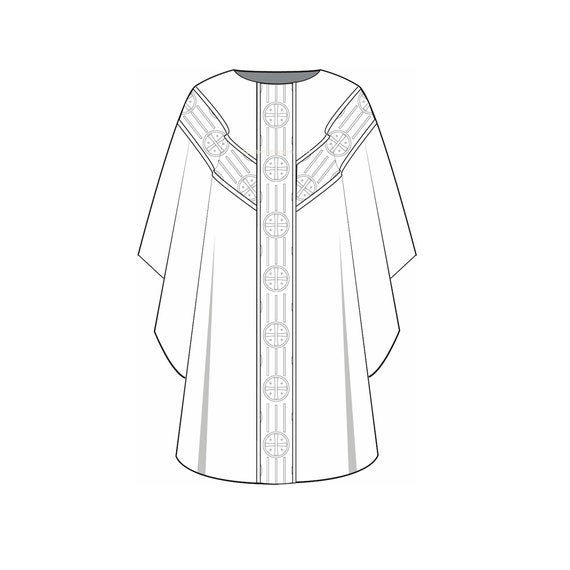The image depicts a detailed, symmetrical, black and white line drawing of a traditional religious robe. The robe is primarily white and extends down to the hem with a striking unique design. This design features a decorative vertical stripe of fabric, running from the neckline to the hem, adorned with seven evenly spaced circles. Each circle is quartered by lines and contains a dot in each segment. Additionally, the fabric pattern emerges one-third down the stripe from both sides, tapering upwards towards the shoulders, creating an almost cross-like shape, though the arms of the cross rise diagonally rather than extending horizontally. The illustration appears to be computer-generated, exhibiting precision and symmetry, and suggests the robe is part of a series of similar designs. The sketch implies a ceremonial or religious context, indicating the robe’s use in traditional practices rather than everyday wear. The gown is presented facing directly towards the viewer, appearing as if it is a preliminary draft for a future creation.